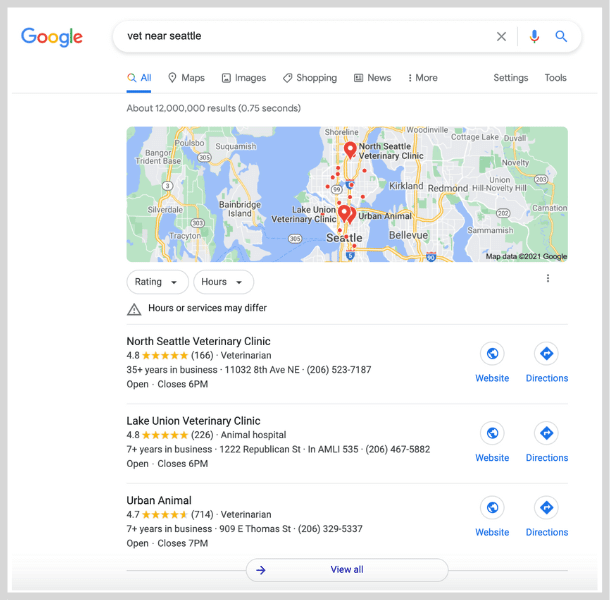The image depicts a Google search results page. In the upper left corner, there is a colorful Google logo. To its right is the familiar search bar, which currently contains the query "vet near Seattle." Adjacent to the search bar are the interactive options: an 'X' to clear the query, a microphone for voice input, and a magnifying glass icon to initiate the search.

Below the search bar, the word "All" is underlined in blue, indicating the current search category. Other category options are listed as: "Maps," "Images," "Shopping," "News," "More," "Settings," and "Tools." Following this, the search results are summarized with the text "About 12,000,000 results (0.75 seconds)," showing the efficiency and vastness of the search.

A large map of the Seattle area occupies a significant portion of the screen. The map visually differentiates between regions with blue areas, yellow-highlighted streets, and red dots marking specific locations. Notable veterinary clinics pinpointed on the map include North Seattle Veterinary Clinic and Lake Union Veterinary Clinic.

Below the map, the search results list detailed information about local veterinary clinics. The first result highlights North Seattle Veterinary Clinic, which has a 4.8-star rating signified by yellow stars along with clickable options to visit the clinic's website or get directions. The second listing features Lake Union Veterinary Clinic, also rated 4.8 stars, with similar options for website access and directions. Finally, the third result is Urban Animal, boasting a 4.7-star rating with 714 reviews, marked by the additional descriptor "Veterinarian" beside its name.